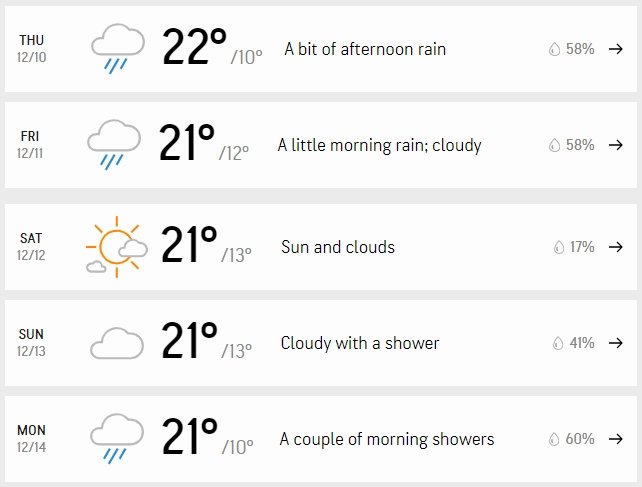This image is a detailed weather forecast for the period from Thursday, December 10th, through Monday. On the left side of the picture, the days and dates are listed vertically: Thursday 12/10, Friday, Saturday, Sunday, and Monday. 

The weather for each day is depicted with icons and descriptions:

- **Thursday:** An icon indicating rain, with a detailed description stating "A bit of afternoon rain." The temperature is forecasted to be 22°C with a low of 10°C. The chance of rain is 58%.
- **Friday:** The icon shows rain again with the description "A little morning rain and cloudy." The high is 21°C and the low is 12°C. The chance of rain remains 58%.
- **Saturday:** The weather is partly cloudy according to the icon and described as "Sun and clouds." The temperature stays steady at 21°C with a low of 13°C. The chance of rain drops significantly to 17%.
- **Sunday:** An icon of complete cloudiness with the description "Cloudy with a shower." The temperature holds at 21°C with a low of 13°C. The chance of rain is 41%.
- **Monday:** The icon returns to rain with a description of "A couple of morning showers." The temperature remains 21°C during the day with a low of 10°C. The chance of rain is the highest at 60%.

The image integrates temperatures, weather conditions, and rain probabilities to provide a comprehensive daily forecast.